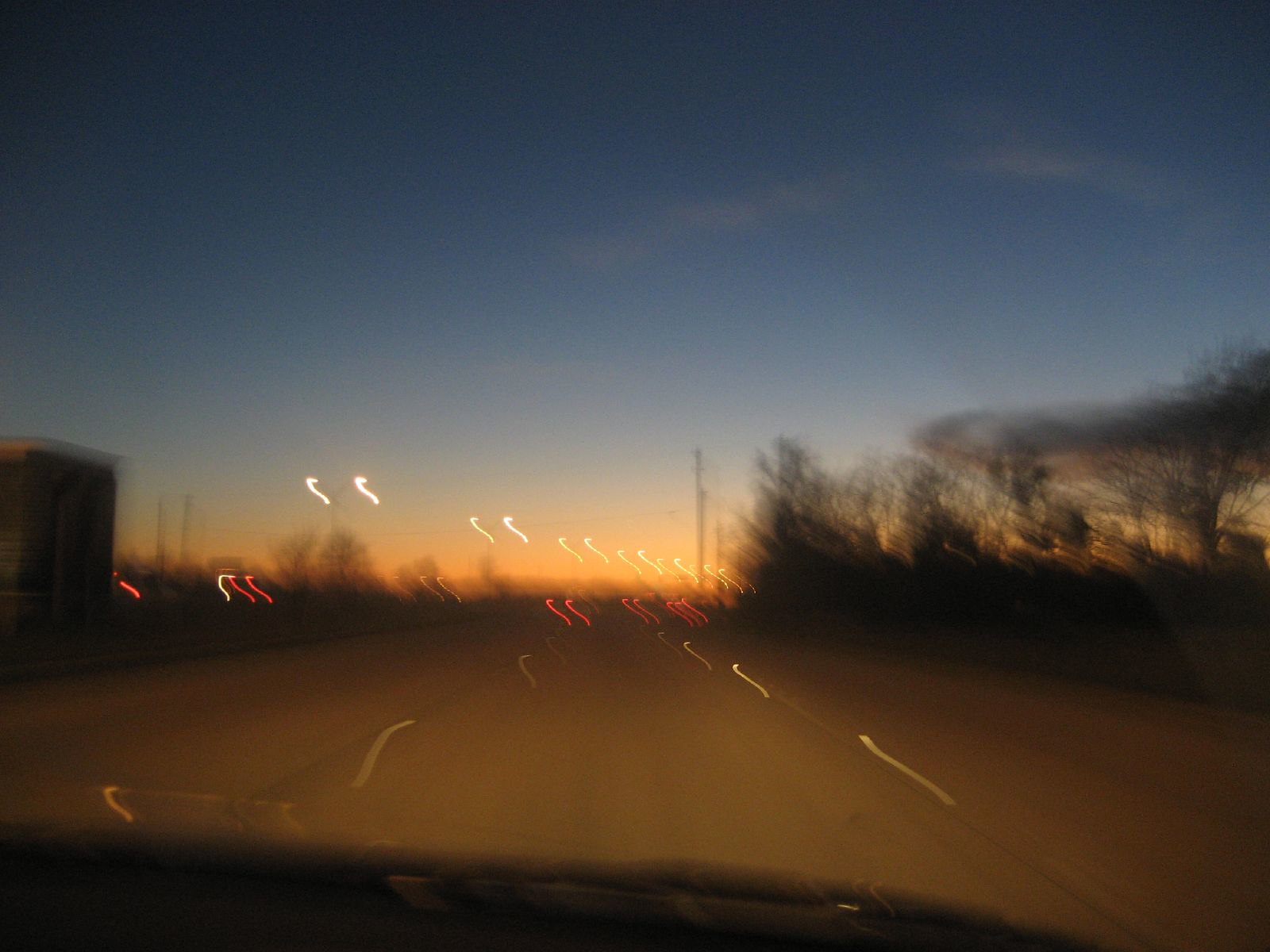This nighttime dashcam photograph, taken at dusk, presents a blurred yet evocative scene. In the foreground, the shadowy top of the dashboard is visible, featuring faint outlines suggestive of windshield wipers. The road ahead is illuminated by winding white lines, reminiscent of serpentine lane markers. To the left, a darkened building emerges, contrasted by a silhouette of trees on the right. Dominating the horizon is a captivating gradient sunset, transitioning from a warm, light orange at the base to progressively lighter blue hues, culminating at the top in a deep, almost navy blue sky. A few wisps of clouds blend seamlessly with the darker blue expanse. Near the horizon, sporadic red squiggly lines and ten white ones—likely depicting the blurred motion of vehicle headlights and taillights—hover ethereally, adding a surreal dimension to this atmospheric capture.